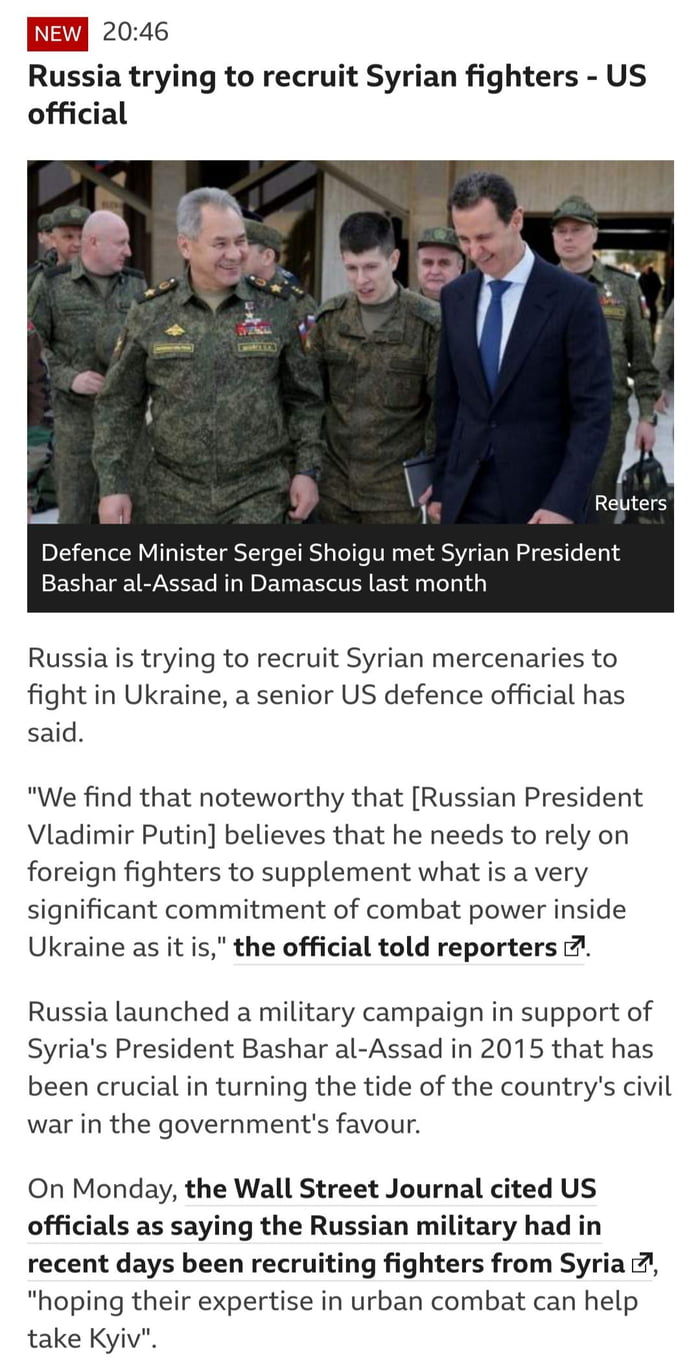An image with a green overlay on a white background features a prominent red rectangle with the word "NEW" in white text and a timestamp "20:46." The story headline reads, "Russia trying to recruit Syrian fighters, U.S. official." Below, a man in a blue suit is pictured alongside army personnel. The caption details a recent meeting where Russian Defense Minister Sergey Shoigu met with Syrian President Bashar al-Assad in Damascus. According to a senior U.S. defense official, Russia is attempting to enlist Syrian mercenaries for the conflict in Ukraine. The official noted, "We find it noteworthy that [Russian President Vladimir Putin] believes that he needs to rely on foreign fighters to supplement what is a very significant commitment to combat power inside Ukraine as it is," addressing reporters. The image also highlights Russia's 2015 military campaign in support of Assad, which played a crucial role in tipping the balance of Syria's civil war in favor of the government.